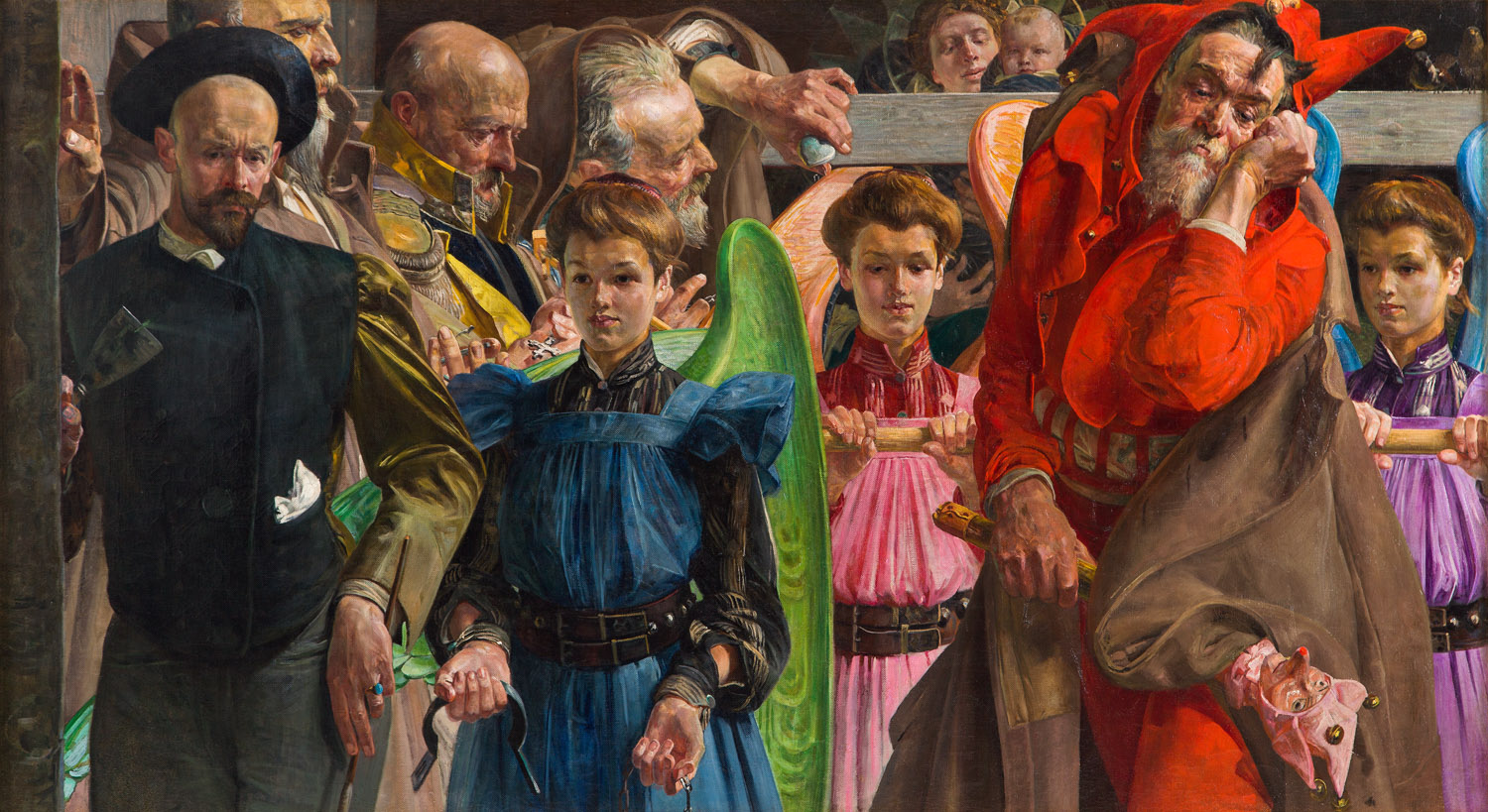The illustration depicts a captivating 18th or 19th century scene featuring various characters adorned in period-appropriate attire. Central to the image are several women who appear to be prisoners, indicated by the leather belts and restraints fastened around their waists and wrists. Each woman is dressed in a distinctively colored smock-like dress – one in blue, another in pink, and the third in purple – and they intriguingly possess large, vibrant wings: green, orange, and blue respectively.

Accompanying the women is a court jester dressed in a striking red suit, complete with a matching red hat and holding a scepter topped with what seems to be the head of a mythical creature or fish. Among the onlookers, there is a man clad in black with a white collar, suggesting he may be a clergy member. Surrounding this dramatic tableau are several other men, either bald or sporting long hair and beards, who observe the scene with a mixture of curiosity and solemnity.

The intricate details of the characters’ clothing and accessories, along with the juxtaposition of historical and fantastical elements, evoke a rich narrative waiting to be unraveled.